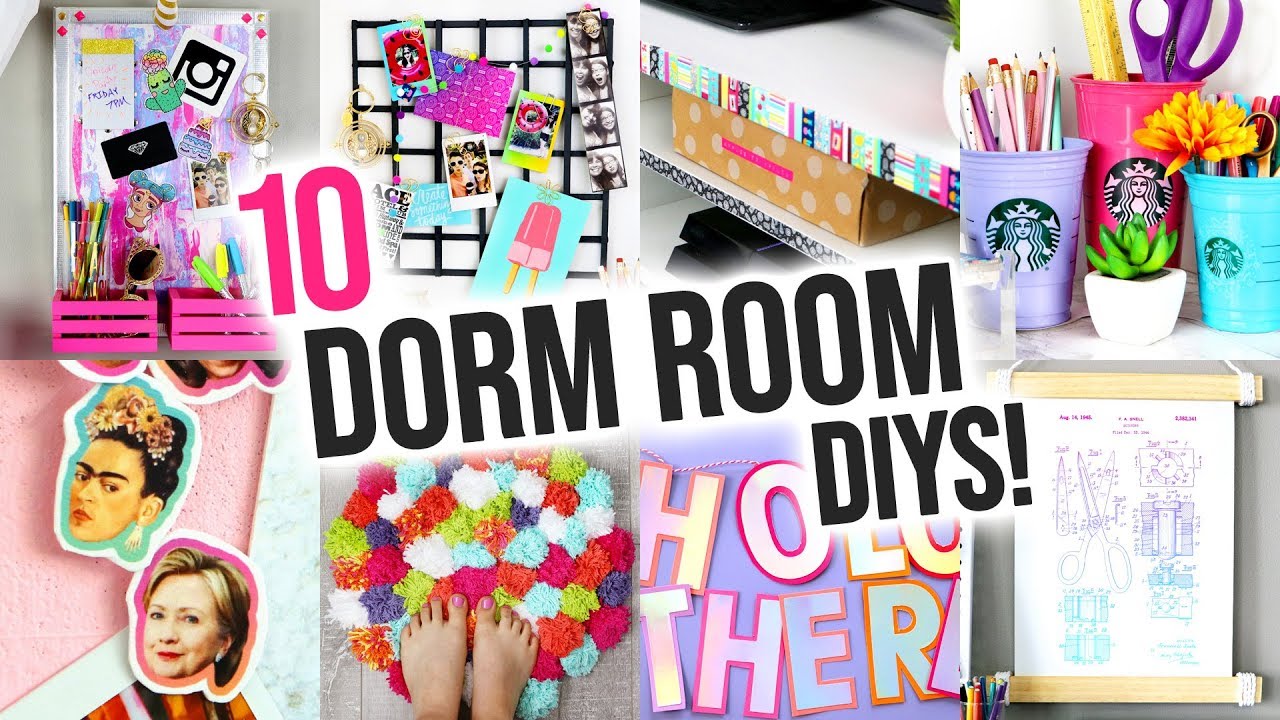This image serves as a vibrant, attention-grabbing Pinterest-style cover photo titled "10 Dorm Room DIYs," with '10' displayed in pink text and 'Dorm Room DIYs' in black text. The collage features eight distinct images, despite the title implying ten projects. The visuals collectively reflect typical DIY ideas for a young, college-aged girl, showcasing creative and colorful decor suggestions.

In the upper right corner, colored Starbucks cups in shades of purple, hot pink, and blue are repurposed as pencil holders, filled with various drawing utensils. The center-left part of the collage highlights a woman adorned with a flower arrangement in her hair, right next to a small but colorful rug, displaying hues such as light blue, orange, hot pink, and purple, possibly DIY'd with fuzzy little balls. Nearby, Hillary Clinton and Frida Kahlo head cutouts add a playful, empowering touch to the decor.

Other images in the collage include a little shelf with pens, highlighters, and notes, and a wire frame intended for hanging small photos or notes. The collection also incorporates various small details such as a ruler, a pair of scissors, and stickers affixed to walls, all of which enhance the do-it-yourself and personalized theme of the dorm room decoration ideas.